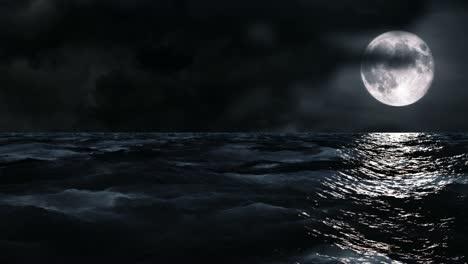The image depicts a striking and possibly artificial night scene over a turbulent ocean, characterized by dark, rocky waves and numerous whitecaps. Dominating the right side of the scene is a large, bright full moon, low on the horizon, casting an intense white light that creates a stark reflection on the water's surface. This light forms a narrow lane running from the horizon to the foreground, distinctly illuminating the otherwise pitch-black waves below. The sky, also intensely dark, features ominous, unnatural-looking clouds that encircle the moon, adding a spooky atmosphere to the scene. Despite its compelling composition, the image appears somewhat artificial, suggesting it might be a composite or created with digital tools such as Photoshop or CGI.